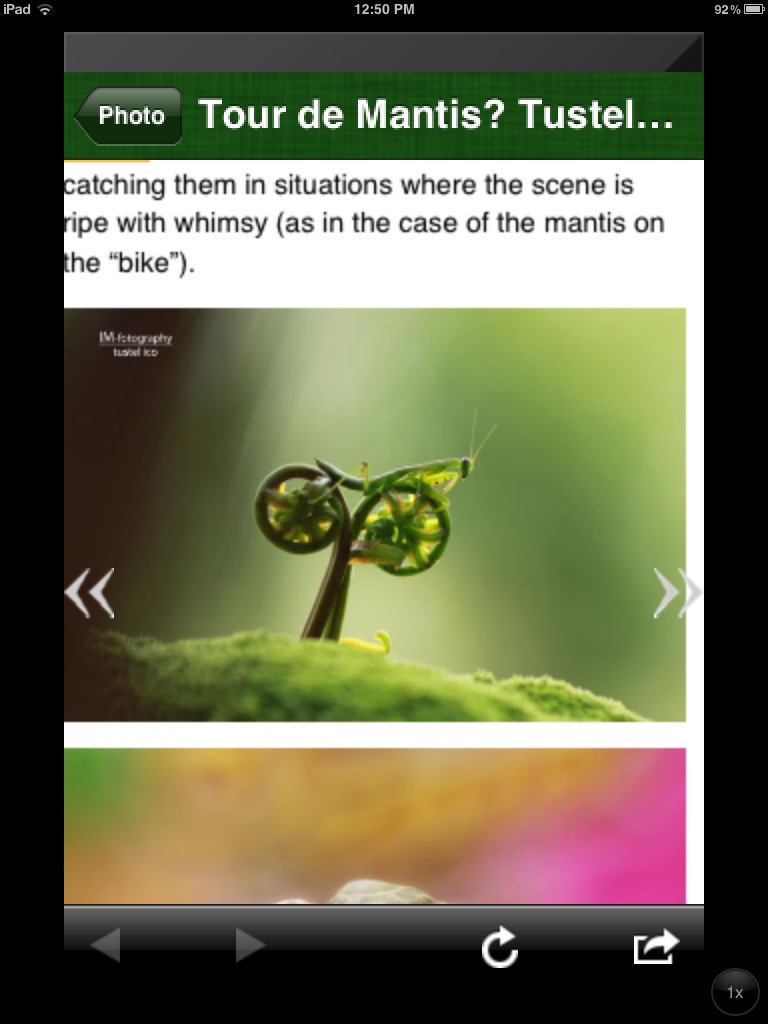This image depicts a detailed screenshot, likely from an iPad or smartphone, with the overall appearance of a cell phone interface. At the top of the screen, the device displays "iPad" in the top left corner, accompanied by a WiFi signal symbol, the time "12:50 PM" in the center, and a battery icon at 92% in the top right corner. 

The central portion features text with a dark green background and white lettering, which reads, "Photo: Tour De Mantis Tussle." This section includes a green arrow pointing left, and beneath it lies a horizontal white band with black text: “Catching them in situations where the scene is ripe with whimsy, as in the case of the mantis on the 'bike.'" 

Occupying nearly half of the screen, there's a landscape-oriented photograph showcasing a praying mantis perched on a green fern, shaped intriguingly like a bicycle, contributing to the whimsical nature mentioned in the text. 

Below this image are partially visible elements with shades of pink, yellow, and green, suggesting another image or part of an interface that is cut off at the bottom. The entire screenshot is bordered in black and includes white navigational buttons at the very bottom. The vivid colors and detailed layout confirm that this is indeed a screenshot from a personal electronic device, capturing a fanciful moment from what appears to be an imaginative article or photo series.